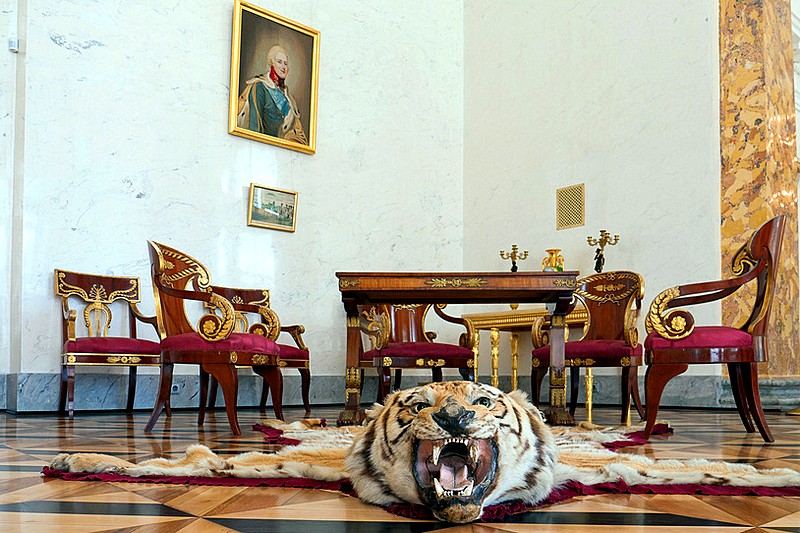The image captures an opulent and elaborate room, reminiscent of those found in castles or luxurious estates. The focal point of the room is a strikingly detailed tiger rug prominently displayed on the intricately patterned wood floor. The rug features the tiger's head, complete with fierce eyes and bared teeth, giving it a lifelike, roaring appearance. Surrounding the head, the tiger's flat skin extends to reveal its iconic stripes.

In the background, a sophisticated wooden table is flanked by several richly upholstered red chairs adorned with gold accents. The chairs feature velvet red cushions and elaborate gold armrests, adding to the room's grandeur. A closer examination reveals at least five of these chairs, arranged around the table.

The walls of the room are painted a light white, enhancing the bright and airy feel of the space. On the left wall, a prominent portrait of a vintage general or dignitary is displayed in a gold frame, with a smaller painting situated directly below it. To the right, there is another piece of artwork and a brown stone pillar that subtly contrasts with the room's overall light theme. Additionally, a golden table is positioned against a wall, further contributing to the ornate decor of the room.